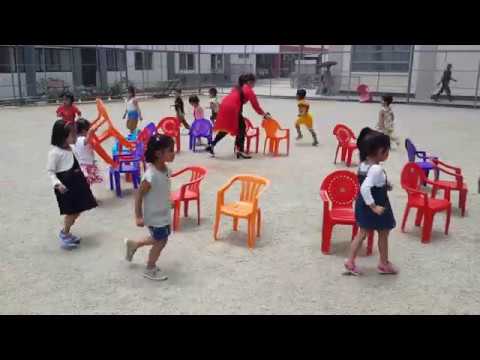In this vibrant and lively image, a group of about ten children is joyfully playing a game of musical chairs in a school playground's courtyard. The children, a mix of little boys and girls, are energetically walking around a circle of small, colorful plastic lawn chairs. The chairs, which are in hues of red, orange, purple, blue, and yellow, form a festive ring on the tan concrete surface. The kids, who are taller than the chairs, are fully absorbed in the game as they navigate around the bright seating. An adult, likely a school teacher, is seen organizing the chairs; she is dressed in a red outfit, black pants or leggings, and black high heels. The background reveals a chain link fence enclosing the area, with buildings partially visible beyond it. The scene is brimming with a sense of fun and community as the children enjoy their playtime outdoors.